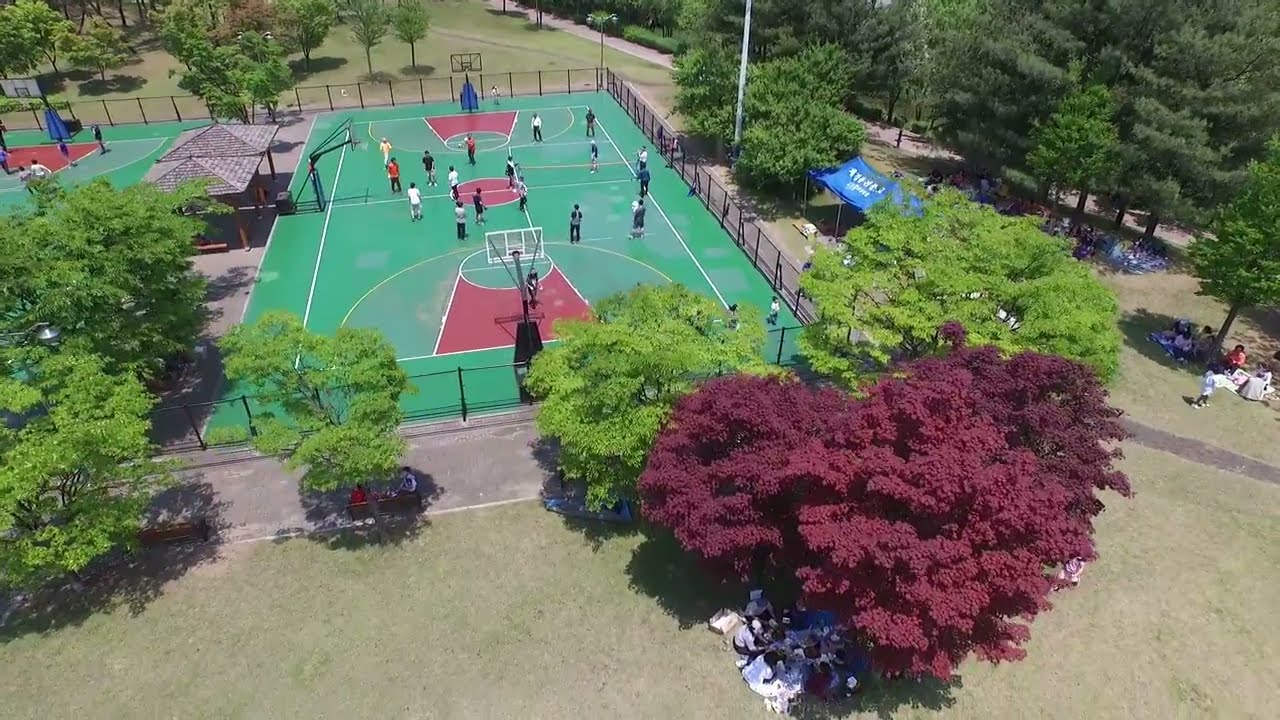This aerial photograph captures a vibrant scene centered around a green and red basketball court, fenced off by a metallic barrier. A lively game is in progress, with players visible in their positions. The court features three basketball hoops, and the red and green paint on the court floor stands out distinctly. Surrounding the court, there is a lush park-like area filled with diverse trees—ranging from light green to dark green, and even a striking red one. The grassy expanse beyond the court is dotted with benches and people. Some individuals are sitting on the grass, seemingly enjoying a picnic, while others are perched in the shade of the trees. To the right of the basketball court, almost out of frame, you can spot a small blue concession stand and a gray pavement pathway. Additionally, a partial view of another basketball court is visible on the left-hand side, where more players are engaged in their own game.